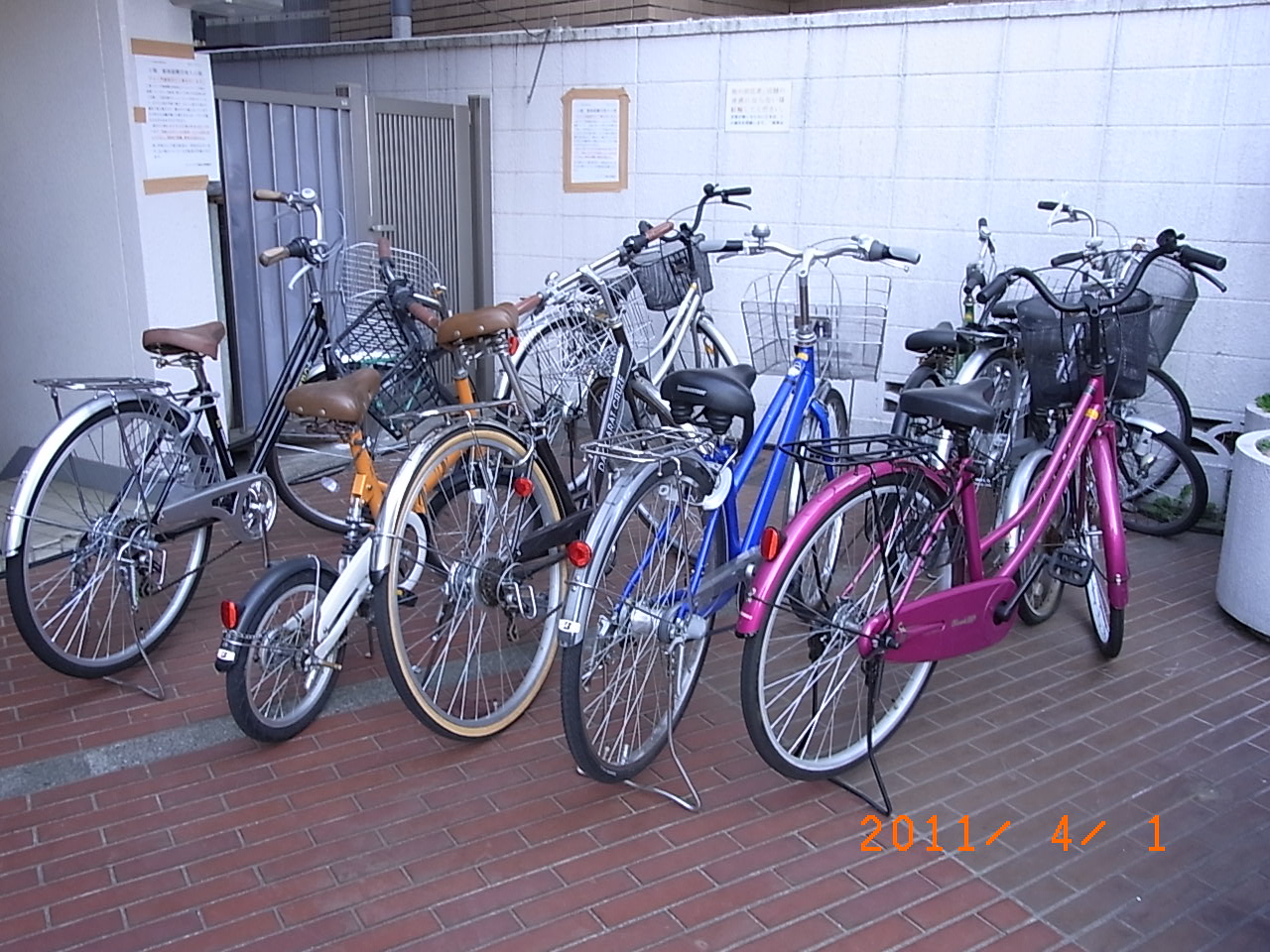The photograph is taken outdoors, featuring a white-painted cinder block wall with a gate on the upper left-hand side, suggesting access to possibly campus housing or an apartment complex. The ground consists of red bricks with white grout. Arranged in the center foregound is a large grouping of approximately nine bicycles of various colors and sizes, predominantly facing the white wall. The most prominent bike on the right-hand side is hot pink with black handlebars and a black mesh basket. Additional notable bikes include a silver, black, purple, and blue one. There are signs on the white wall whose texts are indistinguishable. The bottom right-hand corner of the image displays the date "2011-4-1" in red-orange print, indicating that the picture is somewhat older.